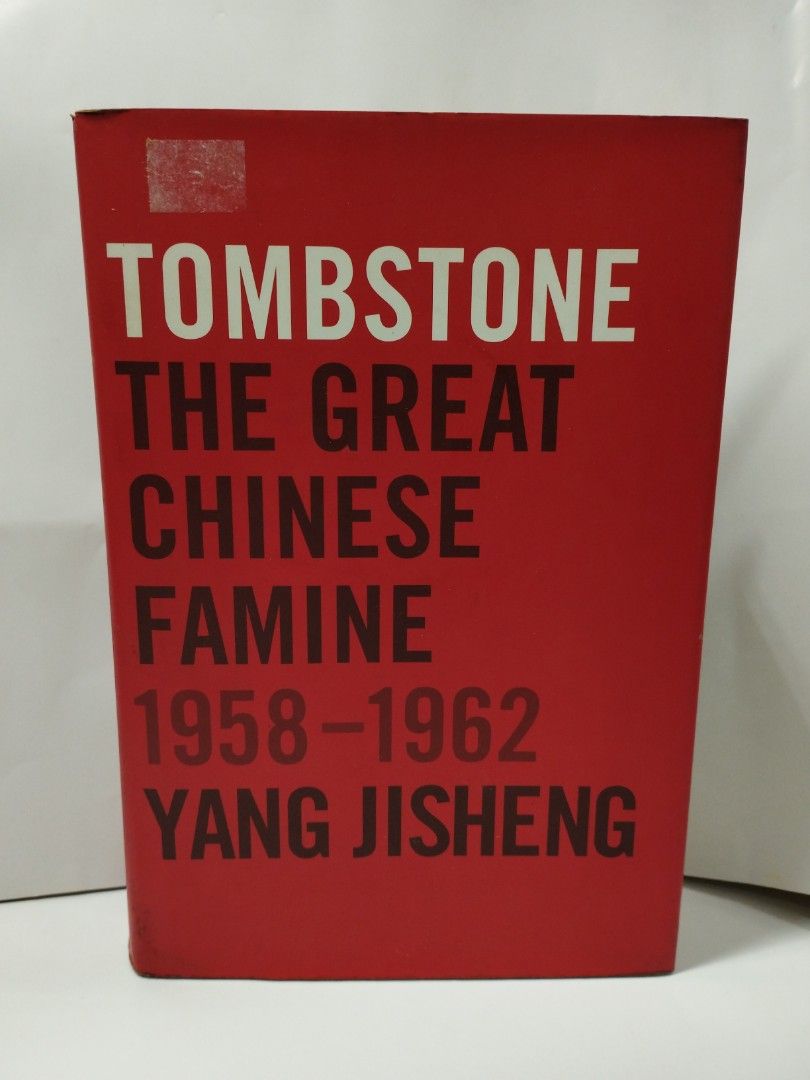The image depicts the cover of a book standing upright against a white background, likely on a white table or platform. The book cover is red, possibly a dust jacket. A notable feature is a rectangular white mark in the top left corner, possibly residue from a removed sticker. The title "Tombstone" is prominently displayed in bold white capital letters below the mark. Directly beneath, in black capital letters, are the words "The Great Chinese Famine," followed by the years "1958-1962" in dark gray. At the bottom, in black capital letters, is the author's name, "Yang Jisheng." The overall photograph is taken from a straight-on angle, emphasizing the book as the focal point, with its shadow cast on the bottom right corner, contributing to the white-dominated backdrop and surface.